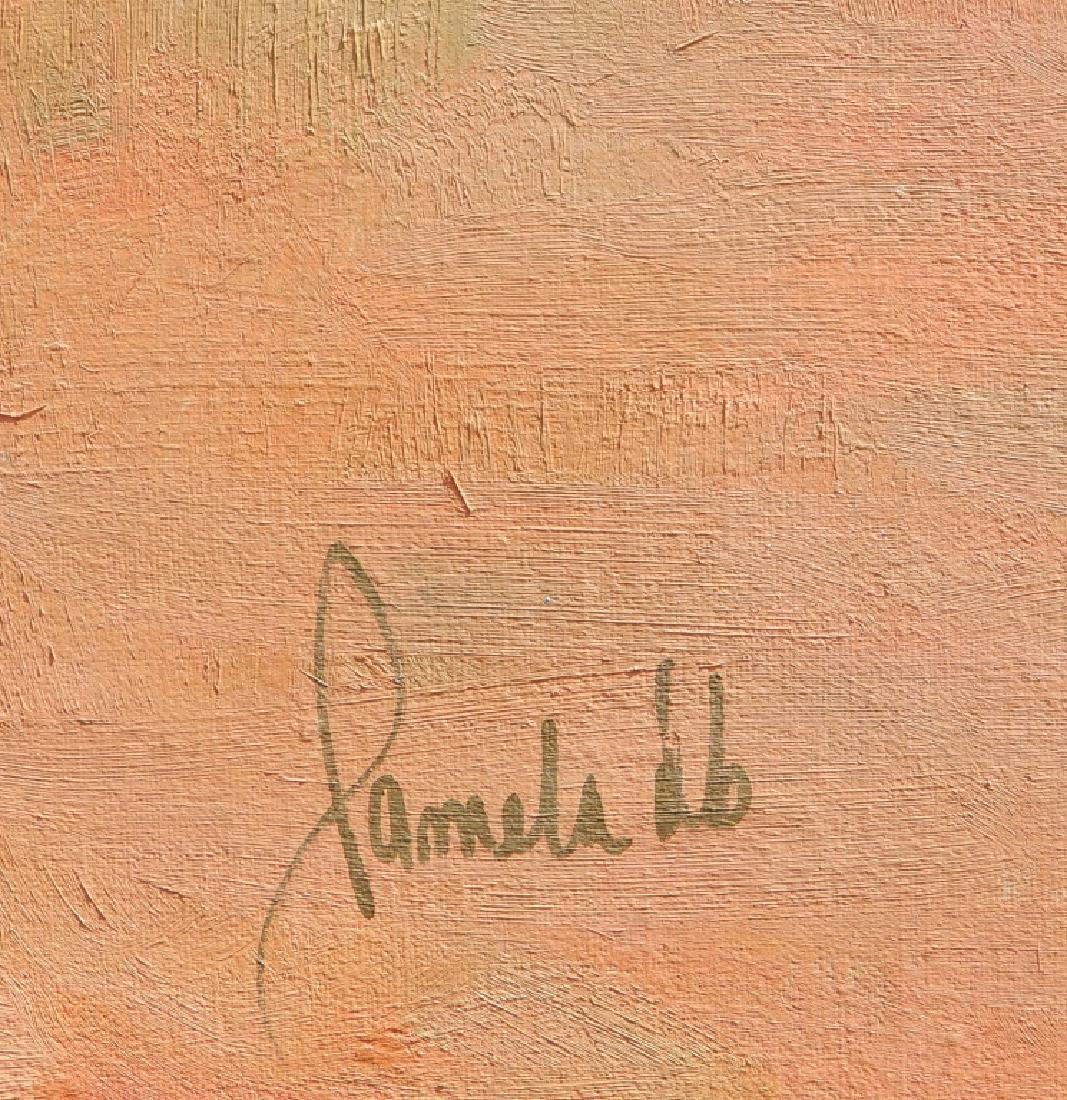The image depicts a textured, stucco-like surface, resembling a rough painting or a section of a wall, with various shades of orange, peach, and beige. The texture includes striations and cross-hatching from noticeable brush marks going in multiple directions, lending a handcrafted quality to the piece. At the bottom center of the image, there is a cursive signature in light brown that reads "Pamela L.B." or possibly "Pamela D.B.," although the exact letters following "Pamela" are not entirely clear. The overall effect is akin to a piece of textured art with a noticeable, personalized signature at the bottom.